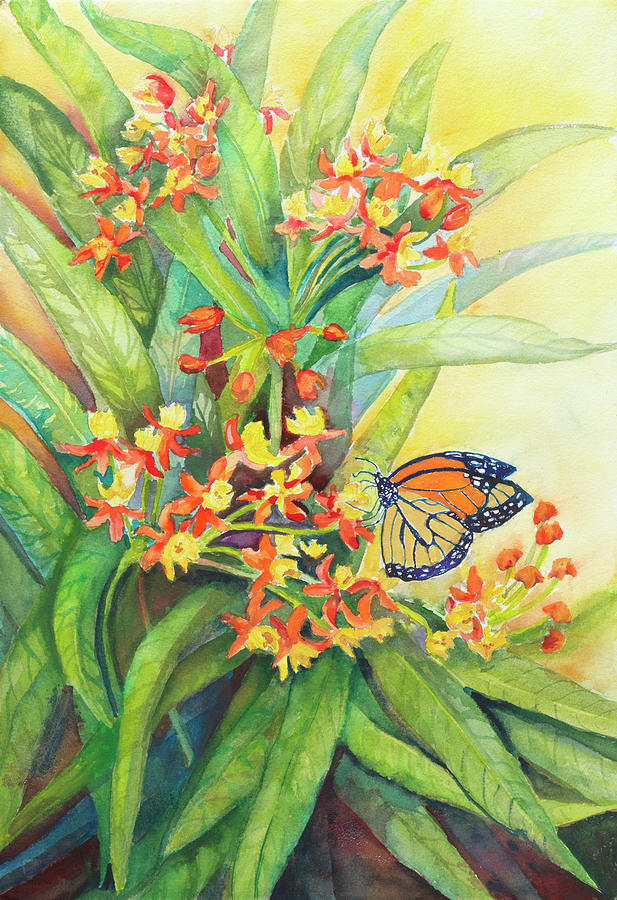The image depicts a detailed painting of a green plant with long, lush leaves. Amongst the verdant foliage, striking orange and yellow flowers with a petal design reminiscent of honeysuckle stand out. Perched delicately on one of these vibrant blooms is a monarch butterfly, characterized by its orange and black wings adorned with white spots and intricate black lines. The background of the painting is a soft blend of pale yellow and white, which gives the impression of sunlight filtering through, enhancing the natural beauty of the scene. At the bottom of the image, beneath the leaves, there's a subtle brownish tone. The overall composition captures a harmonious interplay of colors and elements, creating a serene and captivating portrayal of nature.